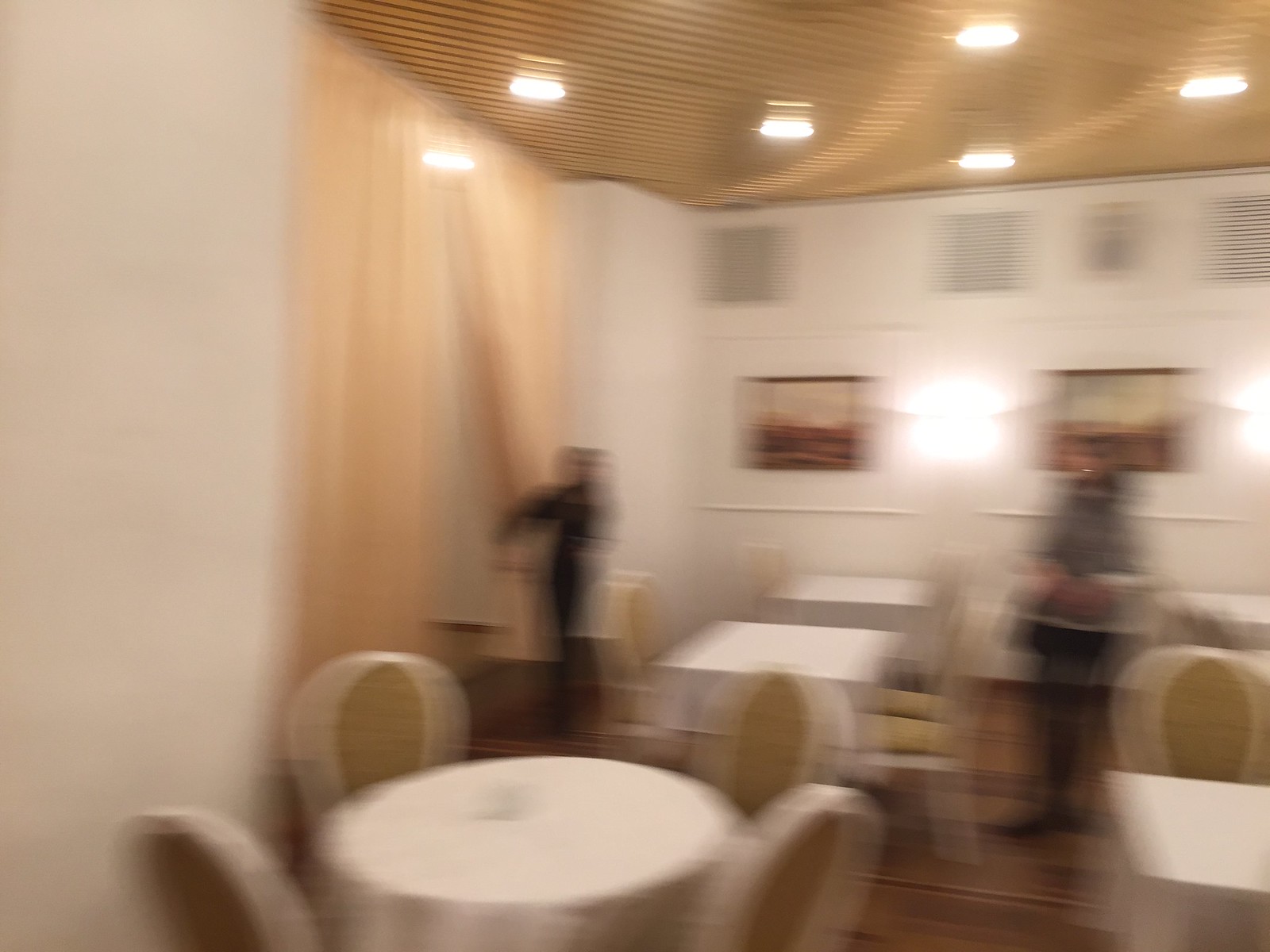This is a slightly blurry, landscape-oriented photograph depicting an elegant dining space, possibly in a high-end restaurant, retirement home cafeteria, or hotel ballroom. The ceiling features goldish-brown parallel lines interspersed with recessed lights, adding warmth to the room. The dining area is furnished with a variety of tables, including a circular table with four chairs in the lower left-hand corner, and at least five other square tables that can accommodate either two or four guests.

The walls are adorned with paintings, adding an artistic touch to the ambiance. On the left side of the image, a person dressed in dark clothing holds open a curtain, seemingly inviting viewers into the room. Another individual stands on the right-hand side, facing forward, but their features are indistinct due to the overall blurriness of the photograph. The scene exudes a formal yet welcoming atmosphere, making it ideal for various upscale dining experiences.